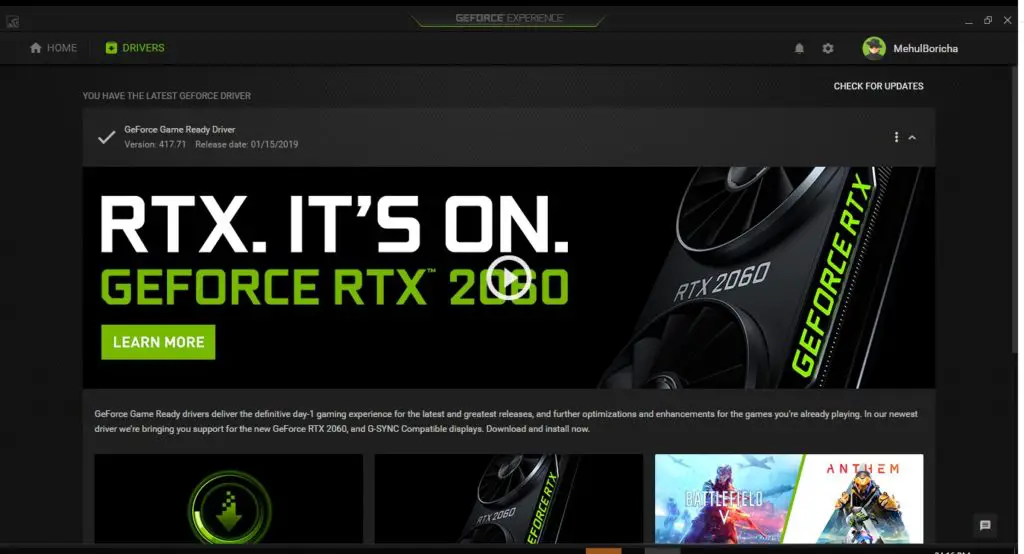The image features a website with a predominantly black background, accented by white and vivid fluorescent green text. It prominently advertises the GeForce RTX 2060, a graphics card designed for gaming enthusiasts. A large image of the graphics card, featuring its cooling fan, takes center stage. Above the card, text reads "GeForce Game Ready Driver Version 417.71," with a release date of January 15, 2019, displayed below. A striking, bright green button labeled "Learn More" invites viewers to explore further information. Although additional text is present at the bottom of the image, it is too small to decipher. In the bottom right corner, game logos for "Battlefield" and "Anthem" are displayed, reinforcing the gaming focus of the hardware. The overall aesthetic, dominated by the black and green color scheme, shares similarities with the branding of Xbox.